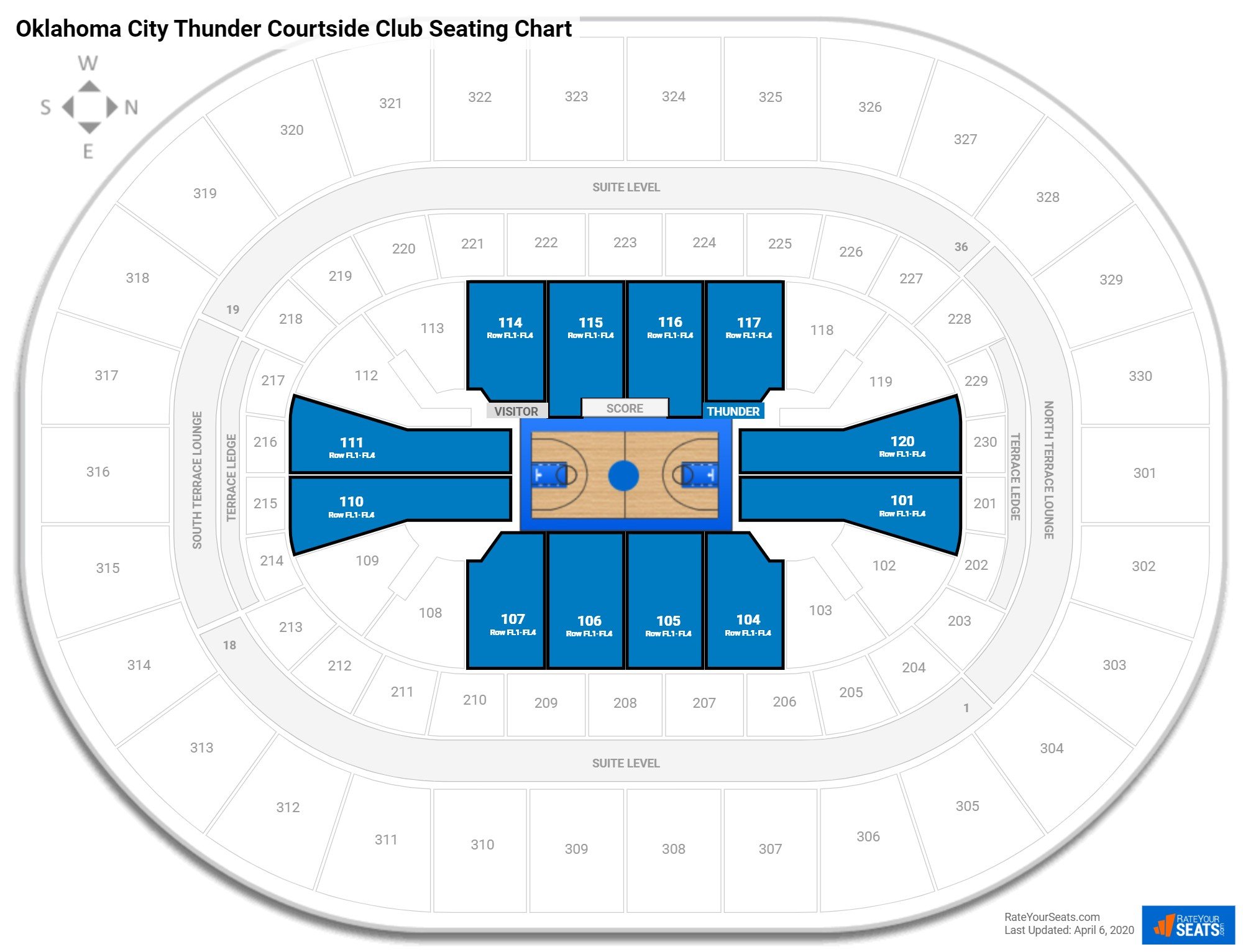Screenshot of Oklahoma City Thunder Courtside Club Seating Chart

This detailed screenshot highlights the seating arrangement for an NBA game at the Oklahoma City Thunder arena. Dominating the top left corner in black text is the title "Oklahoma City Thunder Courtside Club Seating Chart." Directly below, a compass icon illustrates cardinal directions with 'W' for west oriented upwards.

Key sections with courtside seats are distinctly highlighted in blue. Along the top side of the basketball court, these sections include 114, 115, 116, and 117. The right side behind the net features sections 102 and 101, while the left side of the court comprises sections 104, 105, 106, and 107. Positioned behind the left basketball hoop are sections 110 and 111.

The chart also displays all other sections in the stadium, marked in white with grey text, ranging from the 100s to the 300s, and including an intermediate suite level. 

In the bottom right corner, the update information is displayed in grey text: "RateYourSeats.com, last updated April 6, 2020." A blue rectangle adjacent to it features white text reading "Rate Your Seats," accompanied by a logo on the left consisting of three orange bars of varying lengths—a likely representation of the RateYourSeats.com brand.